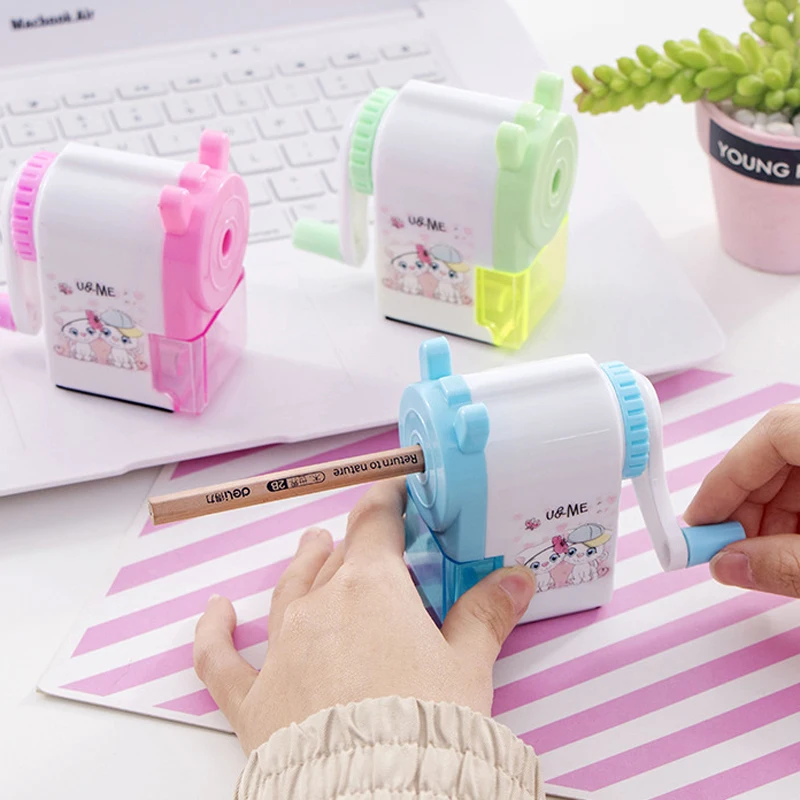In the image, an up-close view showcases three pastel-colored pencil sharpeners, prominently displayed on a white MacBook Air, creating a serene and appealing backdrop. A woman's hands are in the foreground, actively using a light pastel blue sharpener, with a pencil inserted and being turned clockwise. The other two sharpeners—a pastel pink and a pastel green—rest on the laptop's keyboard, each featuring a charming design of a boy and girl cat; the girl cat has a pink bow and the boy cat dons a pastel baseball cap. The text "You & Me" is visible above the cat images. The scene is set on pink and white striped paper, adding a playful touch, while a small potted plant in a pink pot labeled "young" with sprouting leaves occupies the top right corner of the composition, enhancing the youthful and vibrant atmosphere of the advertisement.